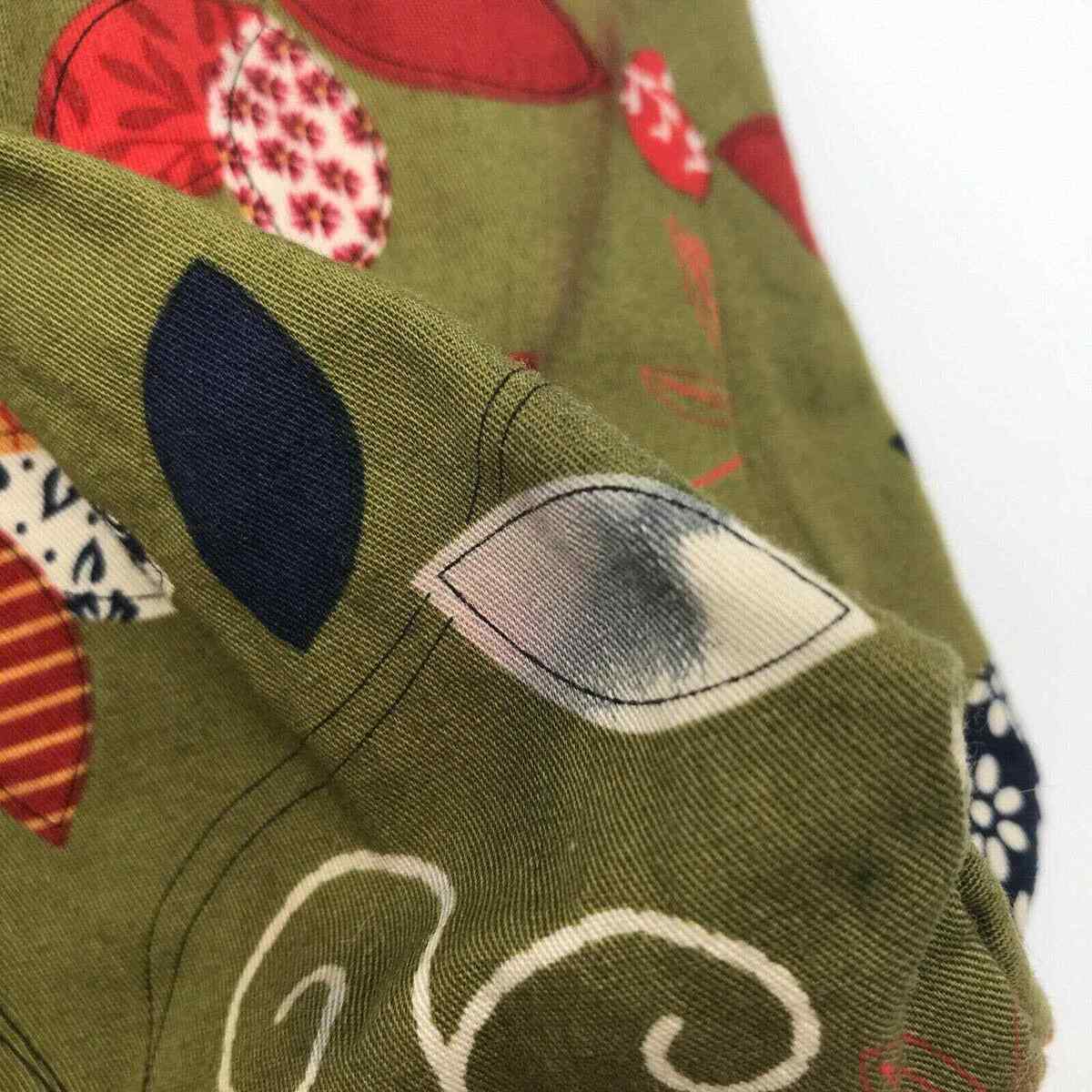This image, most likely a square photograph of approximately six inches by six inches, features a close-up of a green canvas-like fabric, presumably a polyester blend. The fabric, curled up and folded onto itself, obscures much of its larger context. The background, visible only in the top right corner, is a soft, light gray.

The primary focus of the image is the fabric, with its dark mossy green hue and various printed designs. At the bottom, a double twirled white line can be seen, alongside two black lines running from the bottom left corner upwards until they disappear over a fold. Scattered across the fabric are numerous elliptical, leaf-shaped designs in various colors and patterns. These include solid red shapes, a red leaf with a light gray three-leaf print on it, a white leaf with red flowers, a black leaf, and several more intricate designs such as a white leaf with black lining, a white leaf with black polka dots and v-shapes, and a red and orange striped leaf.

Centrally located is a white almond-shaped circle with black stains, which adds to the eclectic patterns. While it's challenging to determine the fabric's purpose, these shapes somewhat resemble eyes, albeit without detailed illustrations. The overall appearance is a rich tapestry of greens, reds, whites, pinks, and blacks, bringing a vibrant and detailed complexity to the fabric's visual narrative.